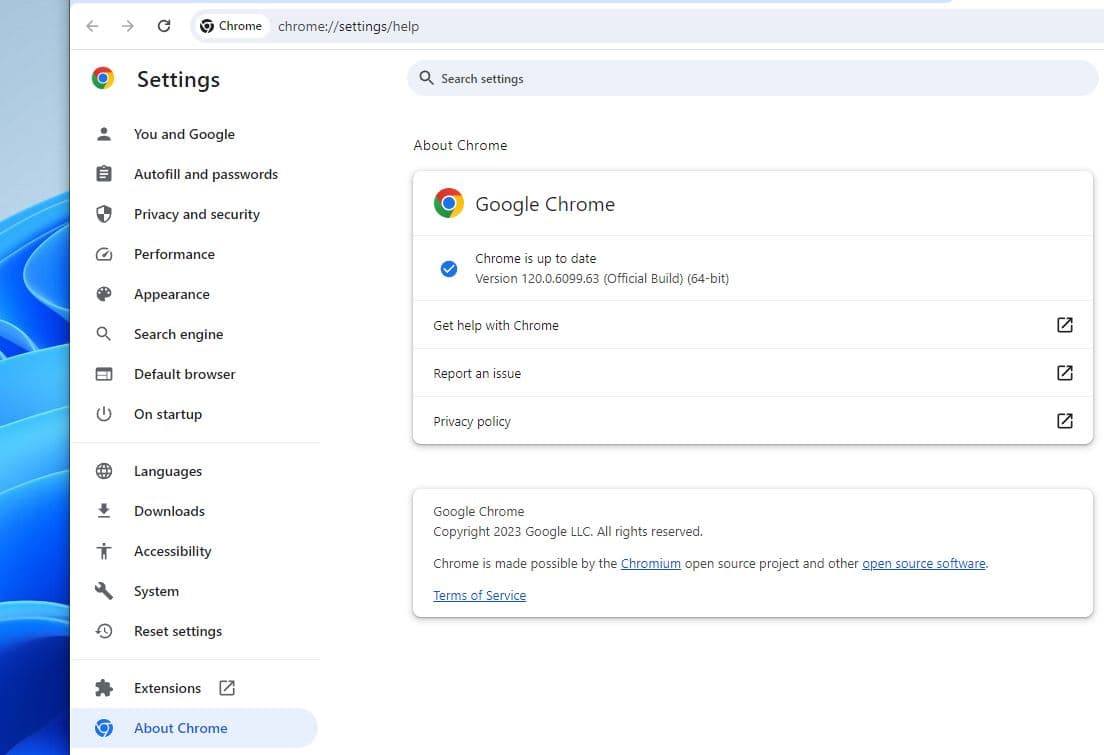A detailed screenshot of a user's computer displaying the Google Chrome settings. On the left side of the screen, there is a comprehensive list of customizable options, including 'You and Google', 'Autofill and passwords', 'Privacy and security', 'Performance', 'Appearance', 'Search engine', 'Default browser', 'On startup', 'Languages', 'Downloads', 'Accessibility', 'System and reset settings', and 'Extensions'. At the bottom of this list, within a small blue box, is the 'About Chrome' section.

To the right, the top of the screen features a 'Search settings' bar. Directly below that, is an informational section about Google Chrome, highlighted by a colorful Chrome logo. The text confirms that "Chrome is up to date" and provides detailed version information: Version 120.06099.63, Official Build, 64-bit. Important links like 'Get help with Chrome', 'Report an issue', and 'Privacy policy' appear underneath.

Further down, another text box provides legal and acknowledgment information: "Google Chrome © 2023 Google LLC, All rights reserved." It notes that "Chrome is made possible by the Chromium open-source project and other open-source software," and provides a link to the terms of service.

On the far left, there's a glimpse of the user's blue desktop background, adding a personal touch to the otherwise technical screenshot. This comprehensive capture clearly highlights the various settings and technical details of Google Chrome.